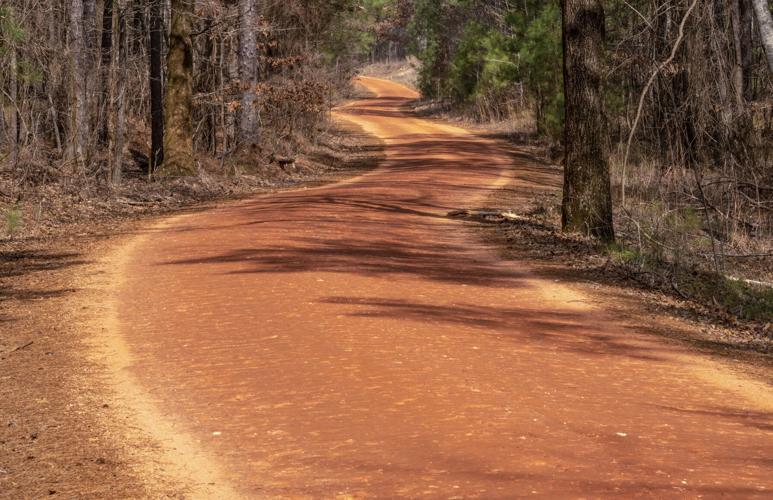The image captures a serpentine dirt path winding through a dense forest. The pathway, mostly a reddish clay color with yellowish borders, zigzags through the scene and seems wide enough for a small car. On both sides of the road are trees, many of which have brown, dead leaves and scattered dead branches, casting intricate shadows on the pathway due to the sunlight that bathes the entire area. However, a striking detail is the presence of green-leaved trees in the distance, adding a touch of vibrance amidst the predominantly brown foliage. This combination of elements highlights a tranquil forest road slowly meandering into the verdant depths.